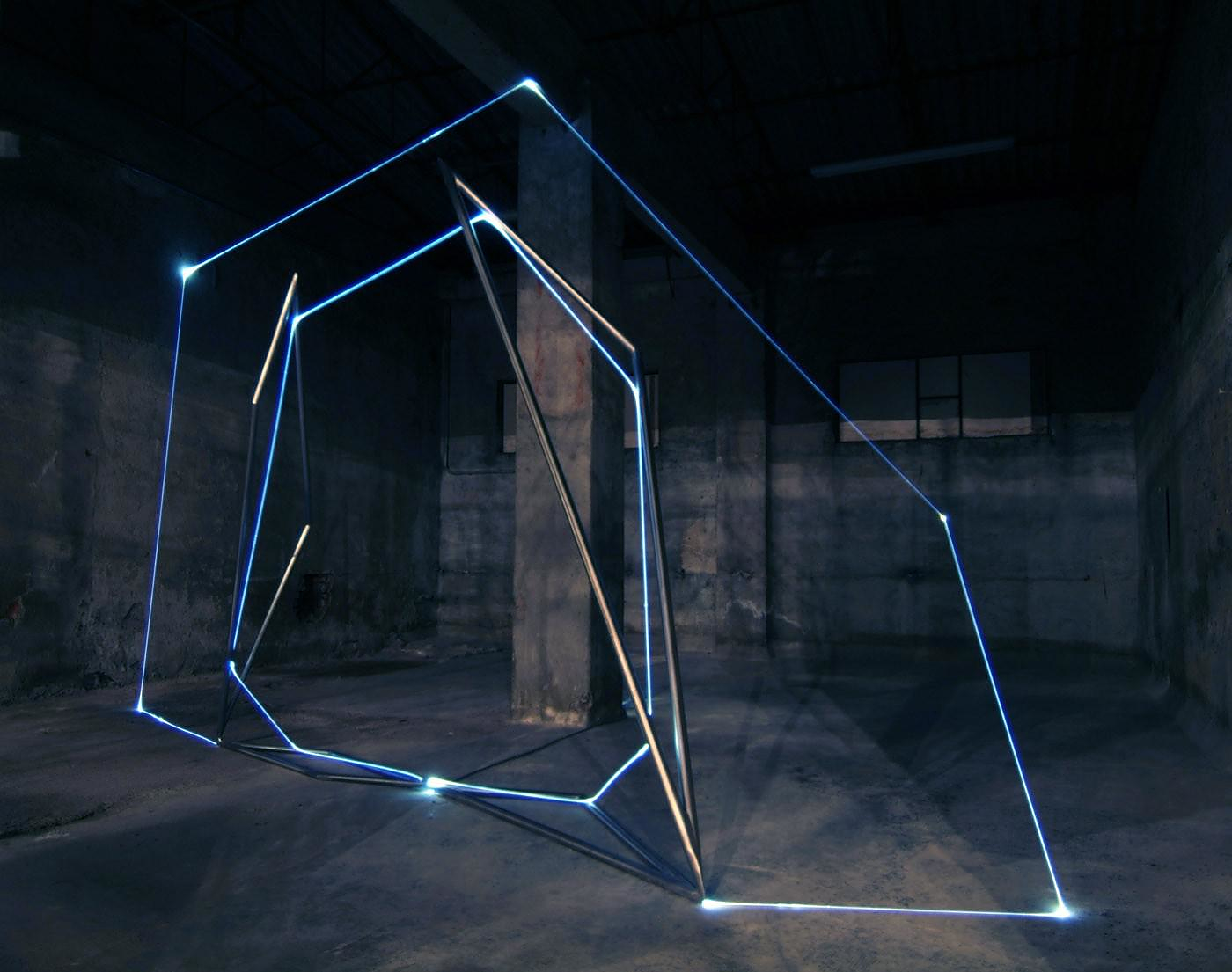The photograph depicts the interior of a dimly-lit, almost empty room with dark gray walls. A central pillar stretches from floor to ceiling. The room's most striking feature is a modern sculpture made of interconnected metallic poles arranged in geometric shapes, such as triangles and hexagons. These poles are bathed in blue laser lights, creating a captivating interplay of light and shadow. The points where the laser lights strike the poles or walls emit a bright white glow, enhancing the futuristic and somewhat surreal ambiance. The minimalistic yet intricate setup, combined with the ambient lighting, lends the room a stark, otherworldly appearance.